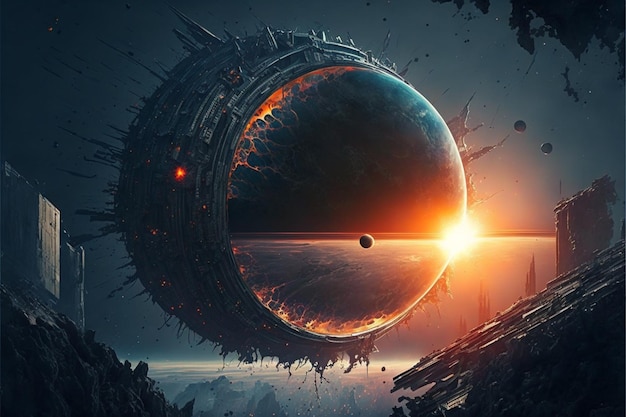The image appears to be a highly detailed, digital, and hyper-realistic rendering of a sci-fi scene set in space. At the center of the composition is a gigantic, spherical spacecraft made of metal. The structure is intricate, with numerous metallic protrusions and elements extending from its surface. One prominent feature is a large, mirror-like lens at the front, reflecting what seems to be the surface of a distant planet along with a smaller planet in the background. This reflective surface also captures the image of a brightly shining sun or star. 

The sphere itself seems to emit a slime-like substance vertically from its body, contributing to the surreal visual effect. The core of the sphere contains a vivid depiction of a horizon with orange hues, and within this horizon lies another smaller sphere, adding depth to the image. Surrounding the central spacecraft are rock-like structures in black or dark gray hues, enhancing the space-bound atmosphere. Additionally, there are square and other geometric shapes interspersed, possibly representing space debris or other spacecraft elements, contributing to the overall complex and mesmerizing scene.